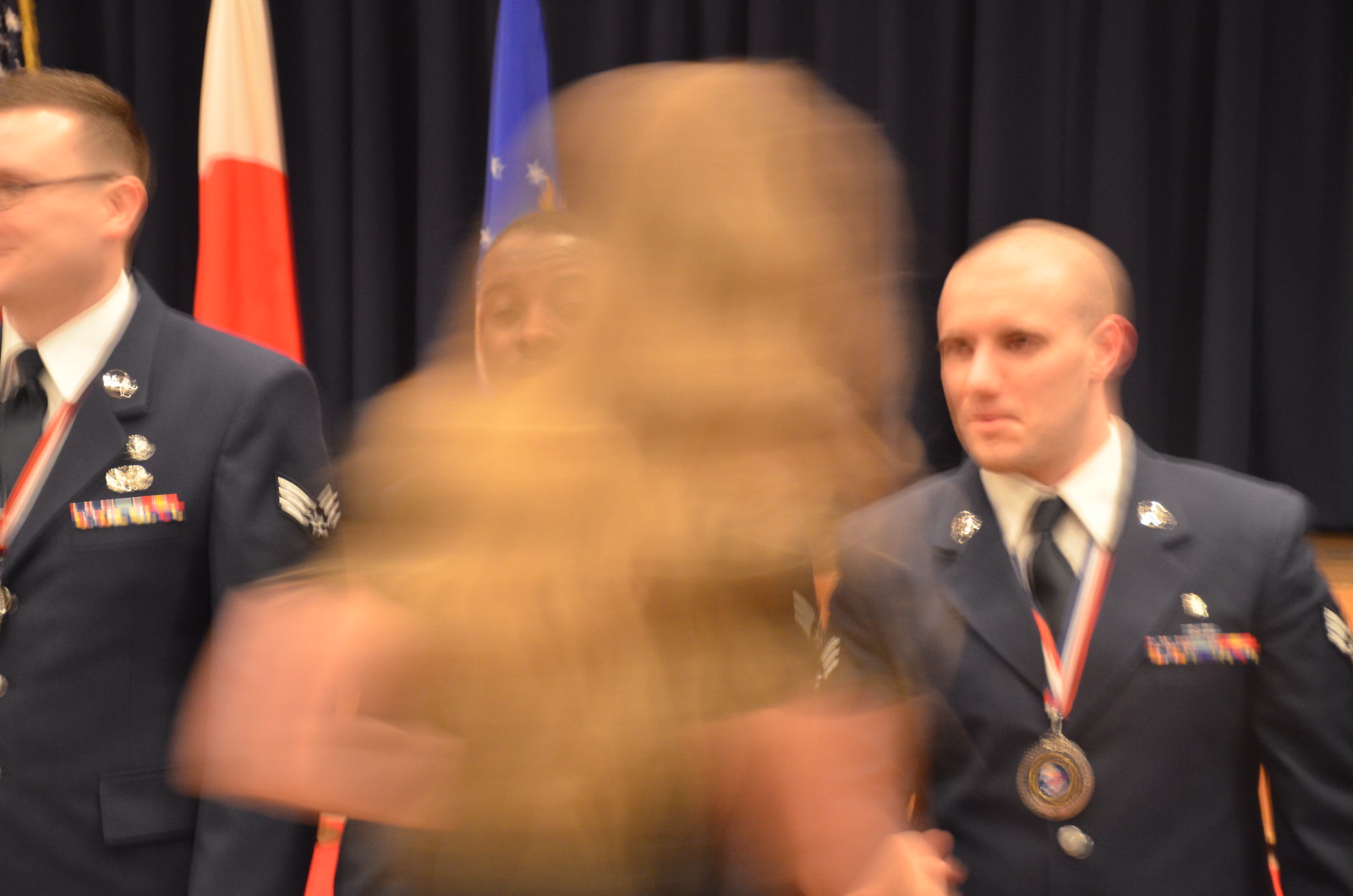The photograph captures a formal military ceremony featuring three men in full military uniform standing on a stage. All three individuals are adorned with various military decorations, including round, gold-colored medals with red, white, and blue ribbons around their necks. They are dressed in white collared shirts, dark blue ties, and buttoned-up blue blazers displaying numerous badges and medals on the right breast. Notably, their jackets bear Air Force wings on the left shoulder. The backdrop consists of a dark blue curtain and two flags. Dominating the center of the image is a large, blurred, semi-transparent figure, possibly someone walking into the shot as the photo was taken, obscuring parts of the men in uniform and making it difficult to discern details in that area. The blur detracts significantly from the clarity of the scene, drawing attention away from the otherwise orderly and disciplined setting.